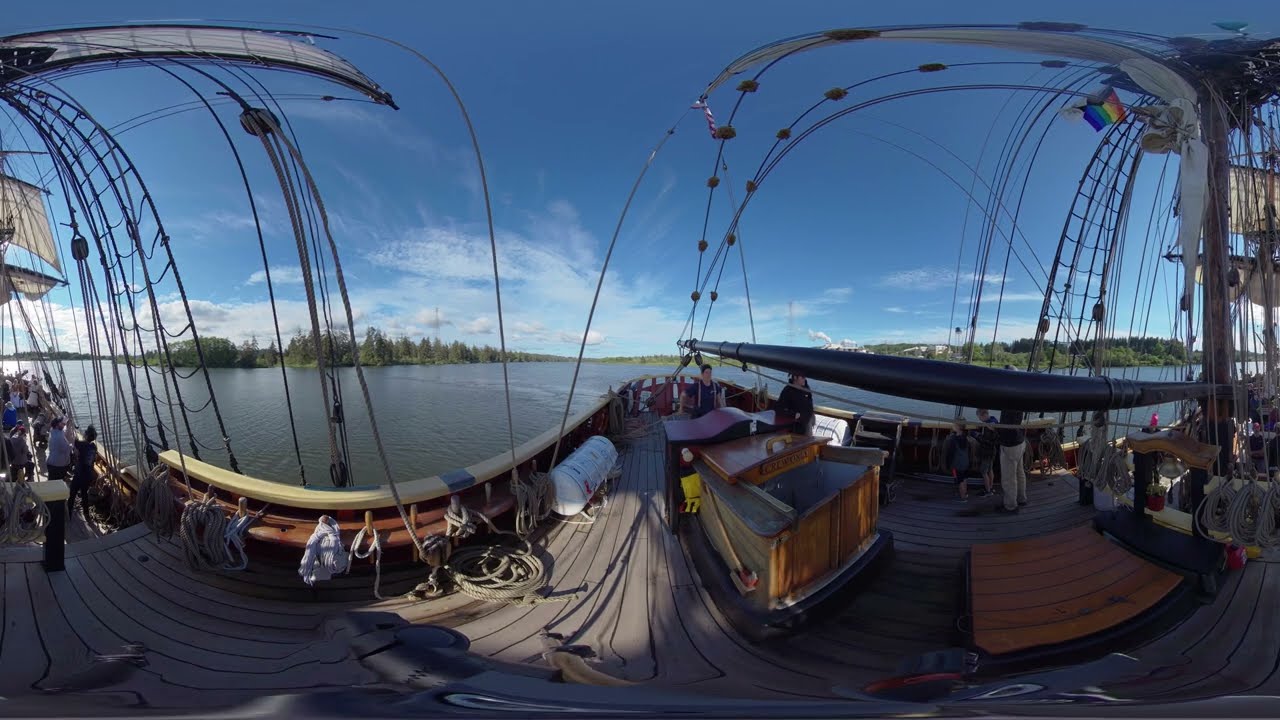The image is a fascinating, panoramic view taken with a fisheye lens from the deck of a large, old-fashioned clipper ship. The perspective is dramatically warped, creating an intensely curved effect on both sides of the image, making the middle appear as if it sinks inward. The deep blue sky above has very few clouds, contributing to the clear day ambiance. Surrounding the boat is a large body of water, possibly a lake, river, or gulf, extending to the tree-lined horizon in the distance, where small pine trees are discernible. 

The boat's deck is replete with details indicative of its age and style. Light brown wooden slats cover the deck, and deeper brown wooden walls rise on either side, crowned with white railings. Numerous ropes are strewn across the deck and hanging from the sides, some coiled and hung on small nubs. On the left and right sides of the vessel, netting reminiscent of classic pirate ships is visible, as well as large, draping white sails. At the top right corner of the image, a small but vivid rainbow pride flag flutters. 

On the deck, although the image is too warped and distant to identify individual features, several people are scattered across the scene. They mingle around the boat, with more on the left side overlooking the water, and a few more spaced on the right. An open hatch to a lower deck is visible, along with what appears to be a white propane tank nearby. The overall scene captures a bustling, nautical atmosphere infused with historical character.